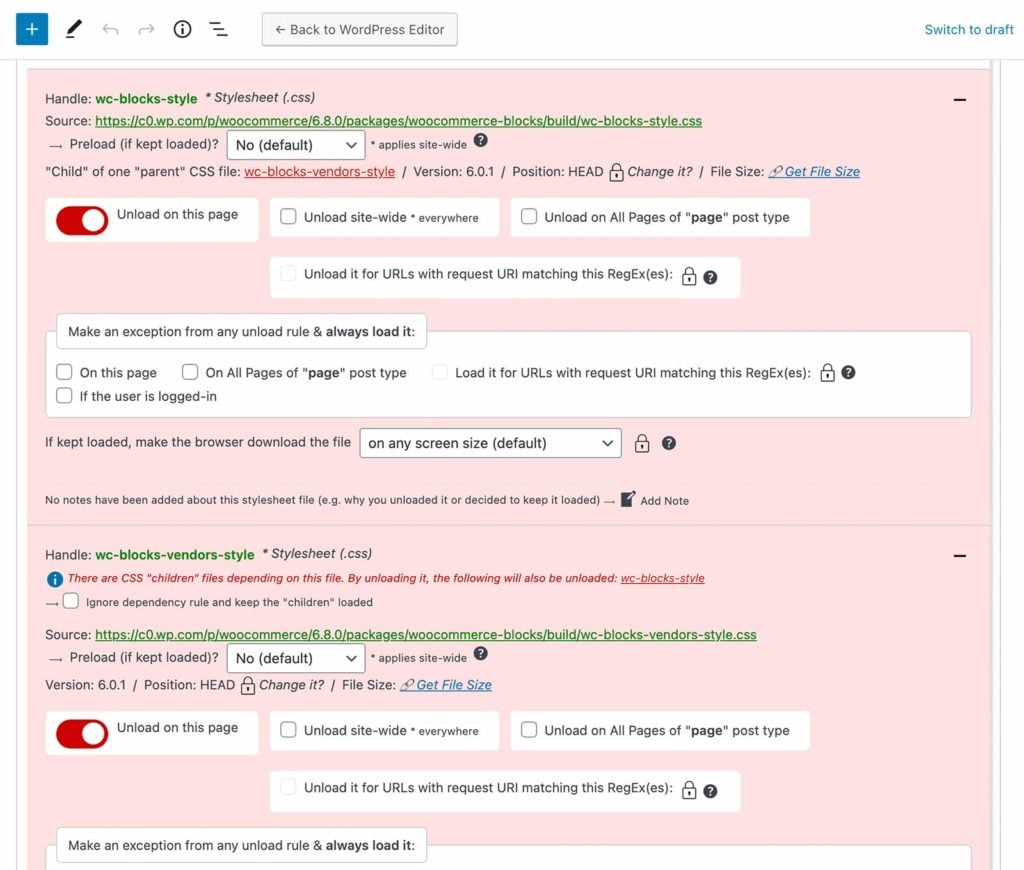Screenshot of an application interface featuring an extensive toolbar and content display elements. The header, primarily white, includes several icons and buttons aligned horizontally. Starting from the left: 

- A blue square with a white plus symbol
- A black, simplified pencil icon at a 45-degree angle atop a horizontal black line
- An arcing light gray arrow pointing to the left
- A mirror image of the previous arrow, pointing right
- A black eye icon enclosed in a black circle
- Three slightly offset black lines, with the top one farthest left and the bottom one farthest right
- A light gray button outlined in medium gray, containing medium gray text with an arrow pointing left followed by "Back to WordPress editor"
- On the far right, blue text that says "Switch to Draft"

Below this header, a thin light gray line separates the toolbar from the main content area. The body of the page has a white background predominantly displaying two pink panes stacked vertically and separated by another thin gray line. 

At the top left of the upper pink pane, black text reads "Handle:" followed by bolded green text "wc-blocks-style." To its right, black text features an asterisk and italicized text "style sheets" in parentheses (.css). Directly below, black text reads "Source:" with an underlined green URL "https://c0.wp.com/p/woocommerce/6.0.0/packages/woocommerce-blocks/build/wc-blocks-style.css."

Additional text continues below on the pink panes, detailing further information.